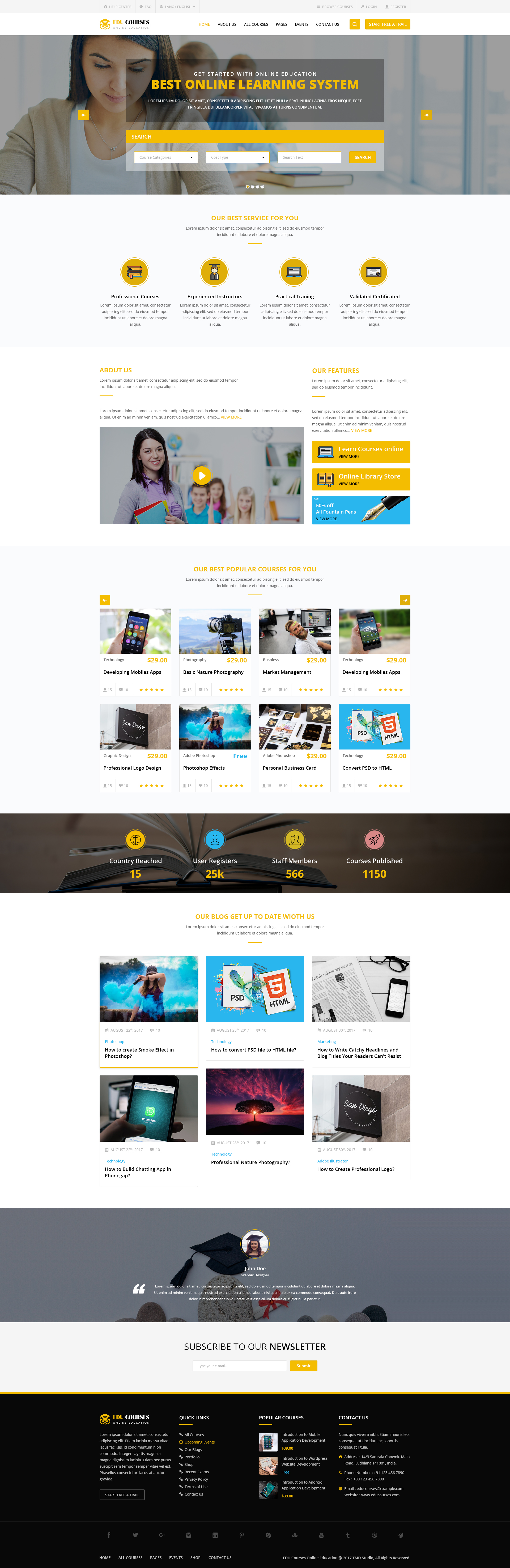This image captures a comprehensive web page for "Edu-Courses," an online educational platform. The navigation menu at the top includes links to "Home," "About Us," "All Courses," "Pages," "Events," and "Contact Us." Also available are options for "Start Free," an "A-Trail," and buttons for "Get Started with Online Education" and "Best Online Learning System."

On the main page, search functionality is provided with fields for "Search Text," "Course Categories," and "Course Type." A prominent section titled "Our Best Service For You" boasts features such as "Professional Courses," "Experienced Instructors," "Practical Training," and "Validated, Certificated" programs. The "About Us" section highlights the platform's future plans, while another section showcases "Our Best Popular Courses For You."

The highlighted courses include "Developing Mobile Apps" at $29, "Basic Nature Photography" at $29, "Market Management" at $29, and "Professional Logo Design" at $29. Each course description is succinct and aimed at attracting students to enroll and take advantage of the affordable, high-quality education provided.